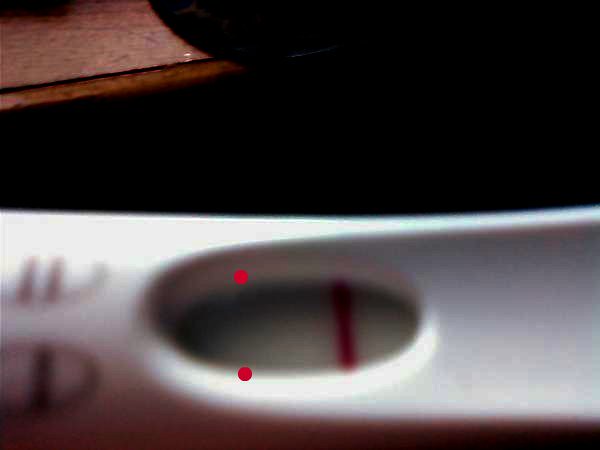A close-up image depicts a blurry pregnancy test, with the focus on a small screen displaying a single horizontal red bar. The precise meaning of this bar is ambiguous, as the test's key indicating the results—typically one bar for not pregnant and two bars for pregnant—is only vaguely visible around the edges. This suggests the test may either indicate a negative result or have yet to be used. Additionally, the image features two red dots at the edges of the test screen, the purpose of which remains unclear. The background above the test is largely dark, making it difficult to discern the setting where the photo was taken.